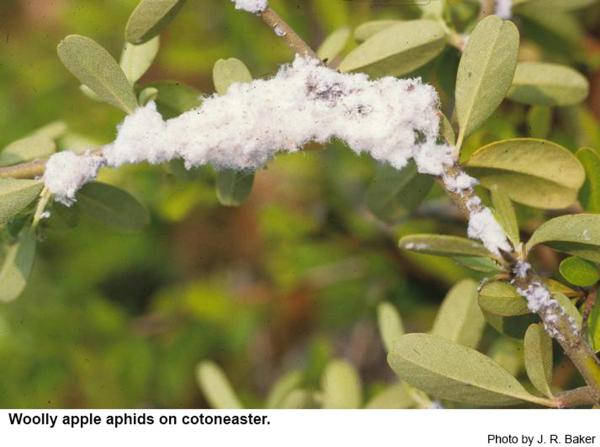This detailed, close-up photograph, taken by J.R. Baker, captures a branch of a plant identified as "cotton ester" prominently showcasing a growth of woolly apple aphids. The branch is enveloped in a cotton-like, matted white substance, which is characteristic of these aphids. Tiny green leaves extend from the branch, adding a delicate contrast to the white covering. The background is an out-of-focus blend of green and red hues, ensuring that the viewer's attention remains solely on the foreground. The image is detailed and vivid, likely intended for use in natural science contexts or educational materials to illustrate the appearance and impact of woolly apple aphids on plants. The bottom of the picture features the text "woolly apple aphids on cotton ester" followed by the photographer's credit, J.R. Baker.